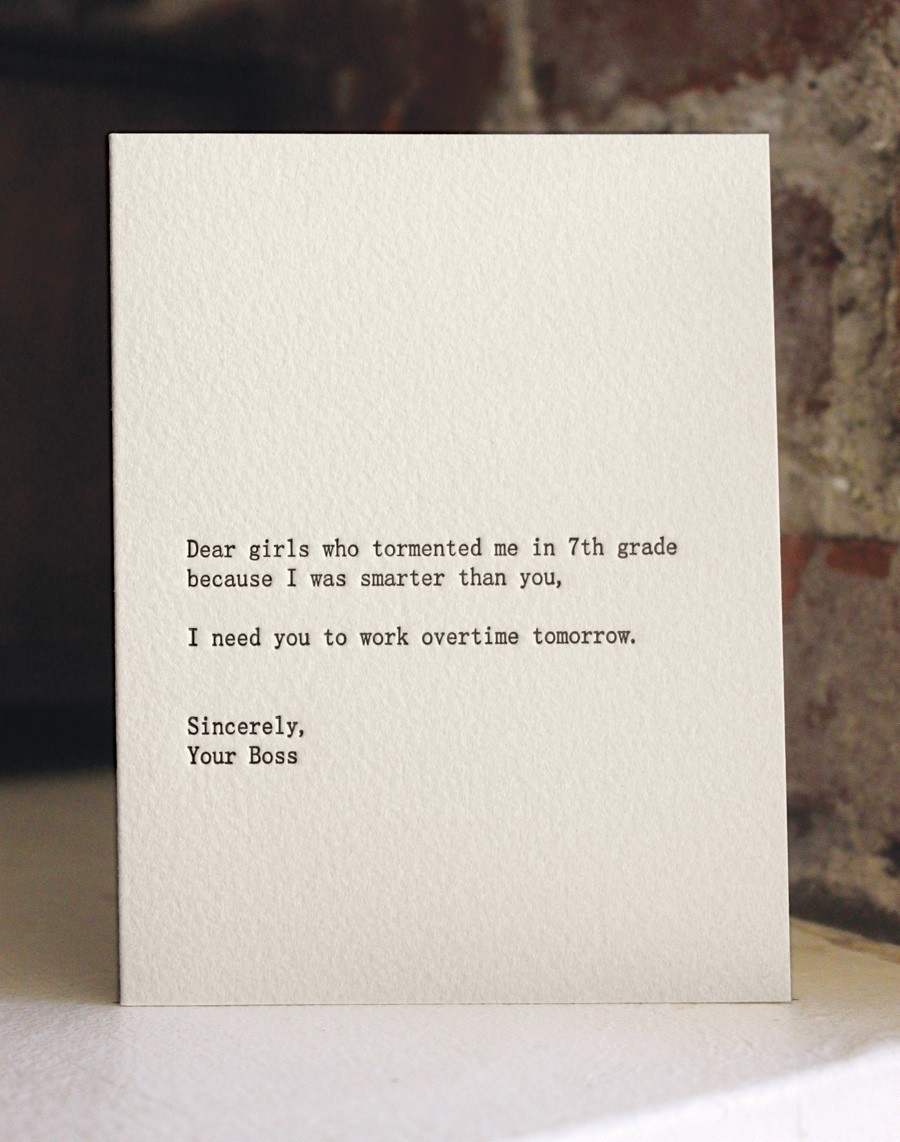The photograph captures a thick, white piece of paper with typed text prominently displayed upright. The text on the letter reads, "Dear girls who tormented me in seventh grade because I was smarter than you, I need you to work overtime tomorrow. Sincerely, your boss," centered on the page. The paper is placed on what appears to be a white surface, possibly a table or a box, in a well-lit room. To the upper left, natural light illuminates part of the scene, hinting at an indoor setting during the day. The background features a distinctive brick wall that mixes shades of gray, white, and red, giving it a somewhat weathered or frayed appearance. The overall composition of the image is clean and detailed, highlighting the contrast between the stark white paper and the varied textures and colors of the brick wall.